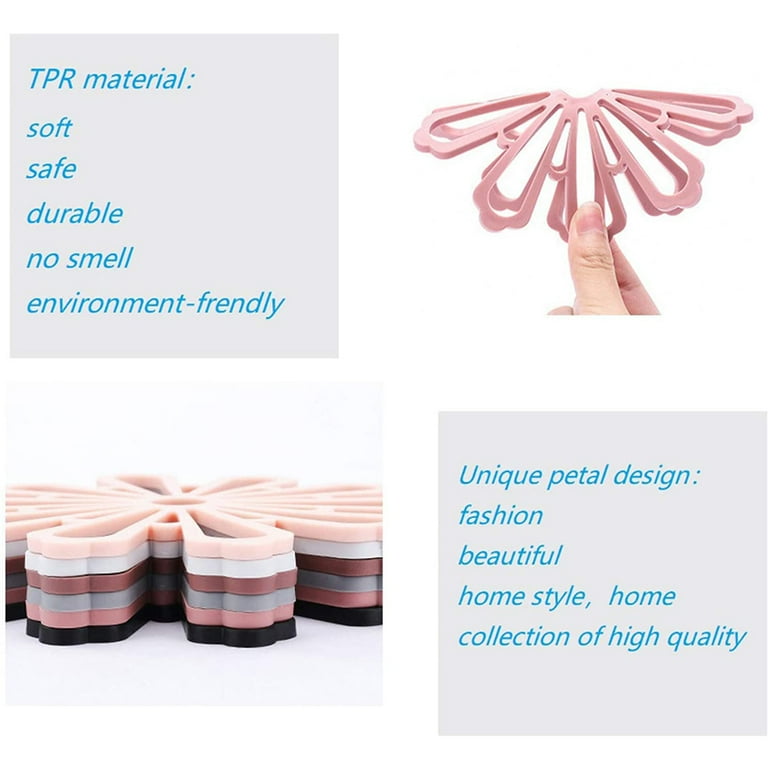The provided graphic appears to be an advertisement featuring two photographs and sections of detailed information. On the left side, a gray box with turquoise (blue) text describes the object as made of TPR material, emphasizing its qualities as soft, safe, durable, odorless, and environmentally friendly. On the right side, another gray box with similar turquoise text describes the design as a unique petal style, highlighting its fashion-forward, beautiful appearance, and suitability for high-quality home collections.

In the top right photograph, a person's hand, specifically the thumb and index finger, is shown pinching a circular, petal-shaped object, demonstrating the material's flexibility. This object appears to be rubberized or soft, akin to a coaster. Meanwhile, on the bottom left, there is another photograph displaying a stack of these petal-shaped coasters. The coasters are arranged in various colors including light pink, white, brown, gray, pink, and black, showcasing their diversity in color options. The petal design of these coasters gives them a distinctive and elegant aesthetic suitable for enhancing home decor.